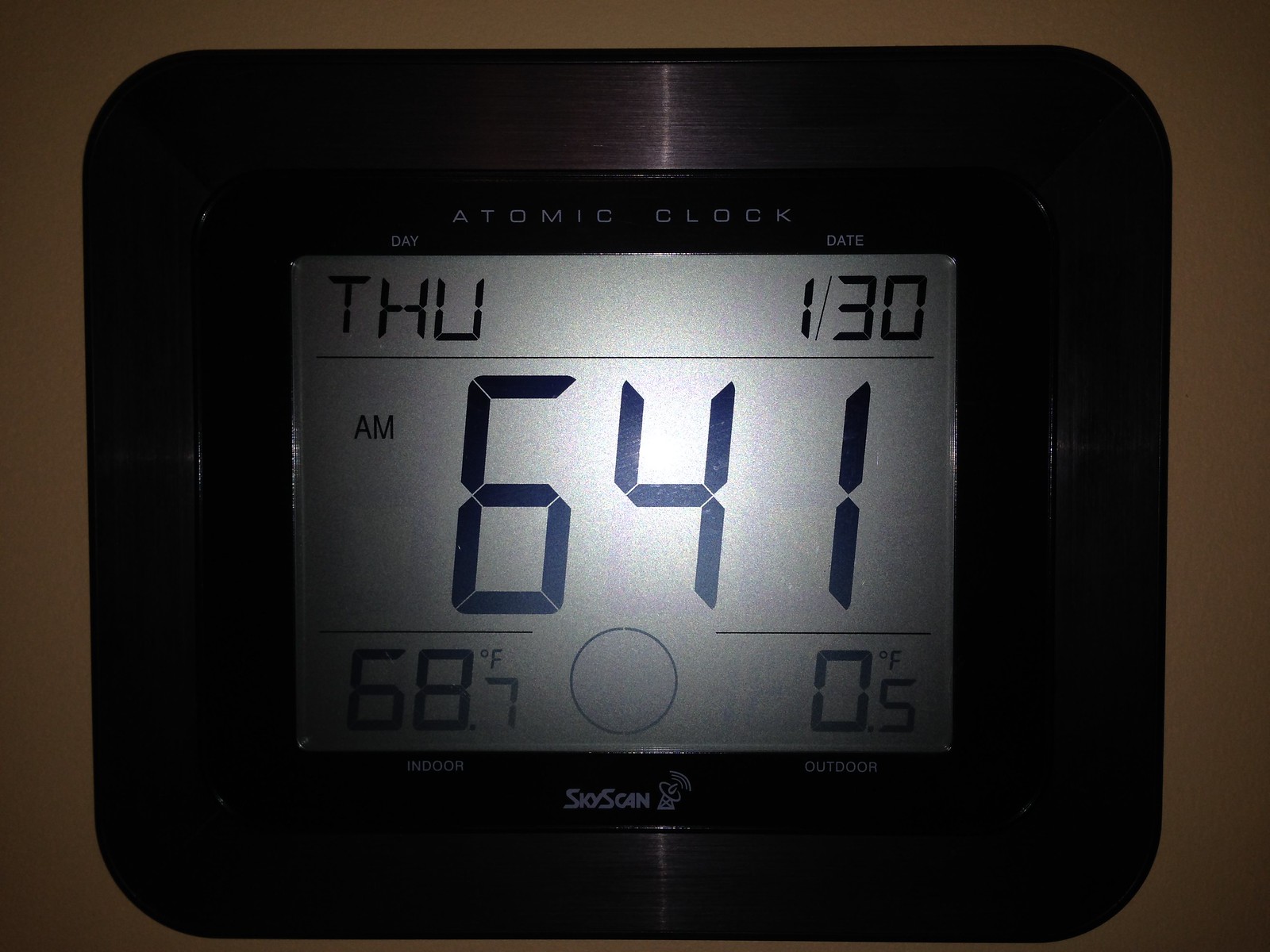Under very low lighting, this photograph captures the face of a digital clock with a rectangular, almost square shape. The clock features a shiny black plastic frame and is mounted on a dark brown surface, possibly a wall. At the top of the clock, the brand name "Atomic Hawk" is displayed in white letters. Below that, two sections indicate "Day" on the left and "Date" on the right. The LCD display shows "THU" for Thursday under Day and "1/30" under Date. Dominating the display, bold seven-segment numerals show the time as "6:41 AM." Beneath the time, a thin horizontal line separates the upper display from the lower section. A small black circle is positioned below the time. At the bottom, the clock provides temperature readings, labeled "Indoor" and "Outdoor." The label "Sky Scan" with an icon of a satellite dish antenna appears inside the frame at the bottom of the clock.